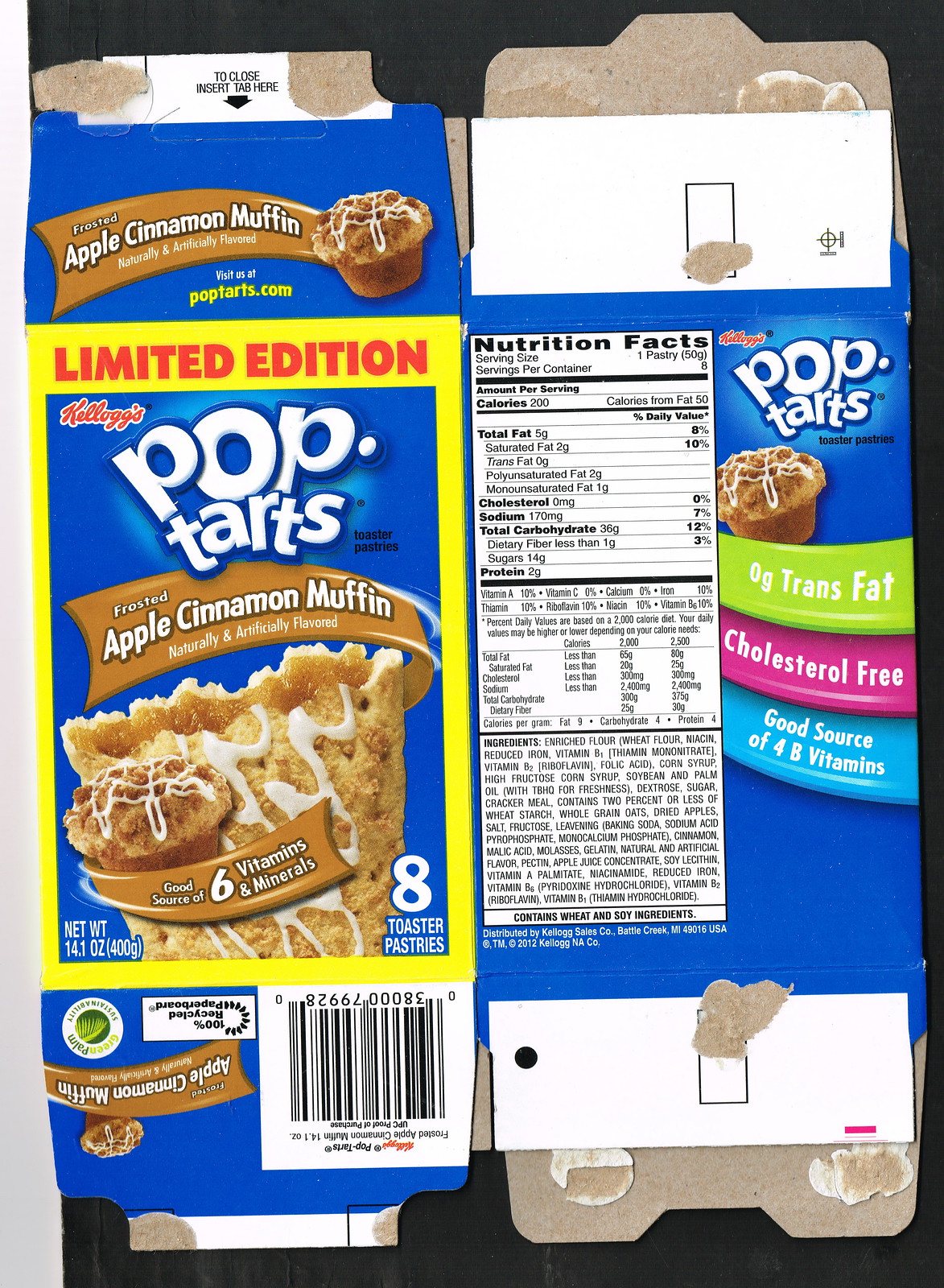The image showcases an opened box of Pop-Tarts, revealing two sides instead of the usual single face. The box is placed against a black background, enhancing its details. 

On the left side, the top flap is predominantly blue and prominently displays the flavor, "Frosted Apple Cinnamon Muffin." The front face of the box features a yellow border with "LIMITED EDITION" written in bold, red capital letters. The main background of this side is blue, with the brand name "Kellogg's" at the top, followed by "Pop-Tarts" and "Frosted Apple Cinnamon Muffin, naturally and artificially flavored." Below this text, there is a vivid image of the Pop-Tart, adorned with white icing drizzles, next to an appetizing muffin. Additional text indicates that the product is a good source of six vitamins and minerals and contains eight toaster pastries. The net weight of 14.1 ounces is also mentioned. The bottom tab includes a UPC code along with the product's name.

The other visible side of the box displays the nutrition facts. It reiterates the product name "Kellogg's Pop-Tarts" and includes an image of the muffin once again. Key nutritional highlights such as "0 grams trans fat," "cholesterol free," and "good source of four B vitamins" are prominently displayed.